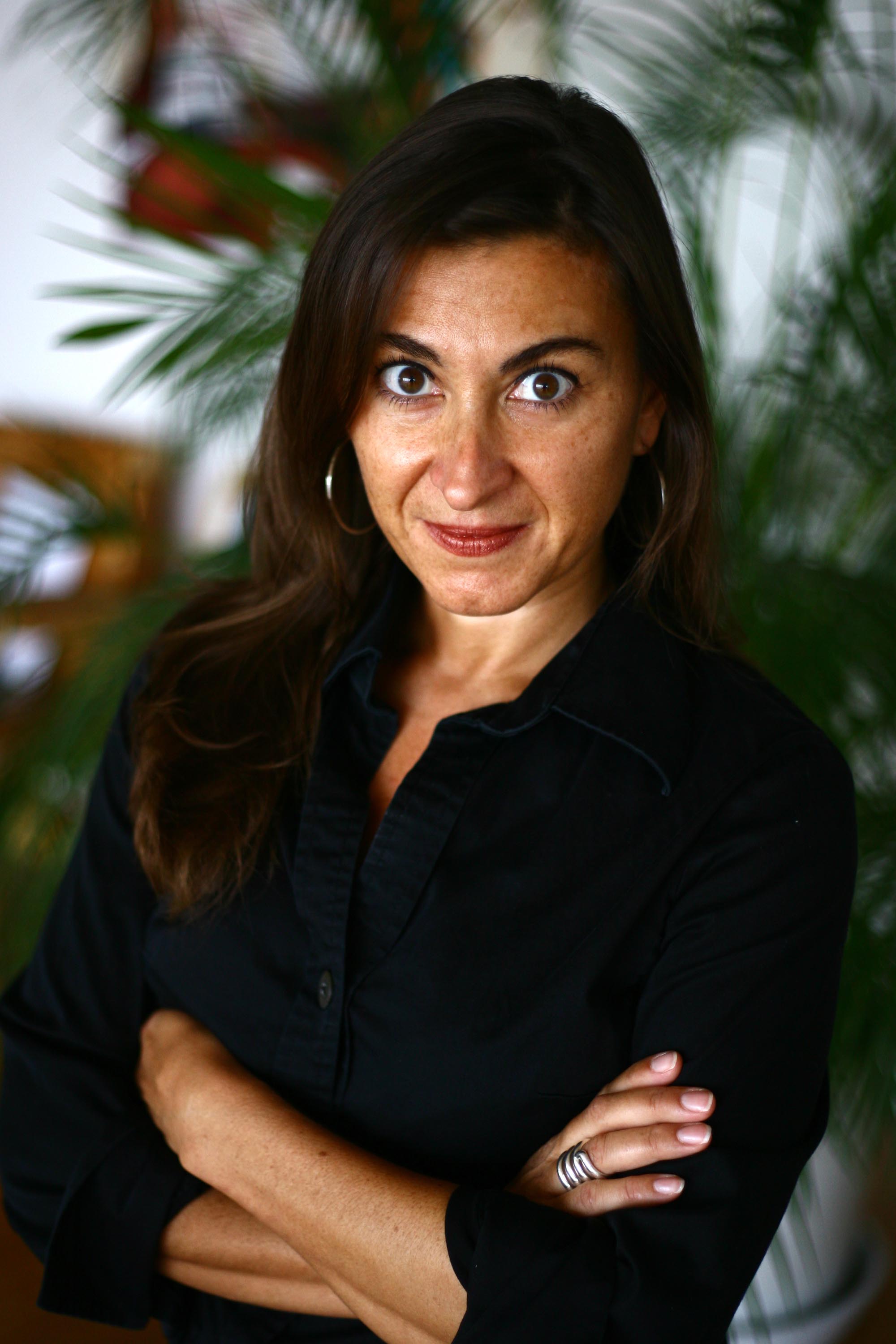The photograph features a woman with long brown hair, parted on the left and cascading down to about her bra strap. She is standing in front of a tall indoor plant, against a slightly blurred white wall adorned with picture frames. She has a tanned complexion with dark, arched eyebrows and wide brown eyes, giving her a very alert and expressive look. She is dressed in a black, button-down shirt with a long folded collar and long sleeves that come down just below her elbows. Her arms are crossed in front of her, revealing groomed and buffed nails, and she wears a distinctive silver ring with multiple loops on her right hand. She also sports large silver hoop earrings and a touch of lipstick. The overall composition and her poised, engaging expression suggest that this could be a headshot for a magazine article.